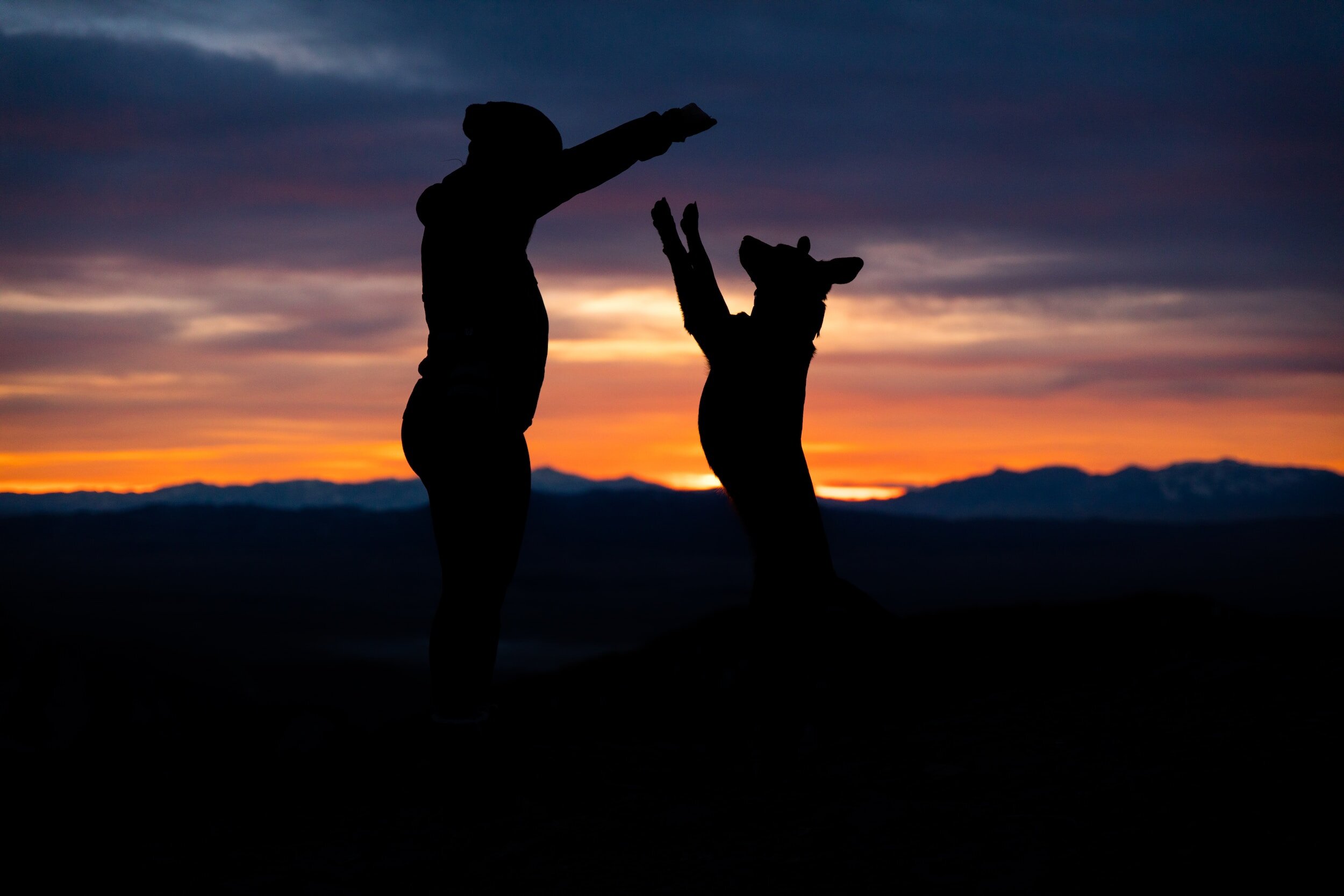This photograph captures a mesmerizing sunset scene with vibrant hues spanning from yellow at the horizon to orange, pink, white, and progressively darker blues as they reach the top. Dark clouds loom overhead, casting a serene, yet dramatic ambiance. The bottom of the image is shrouded in black, with hills silhouetted against the colorful sky. Emerging from this darkness are the shadowy figures of a person and a dog. The person, in side profile, wears a hoodie, hat, and long sleeves, with one hand extended out in front, possibly offering a treat. The dog, which resembles a shepherd, stands on its hind legs with its front paws stretched upwards, its two ears perked up attentively. This moment of interaction between the human and the dog is beautifully set against the stunning backdrop of the sunset.